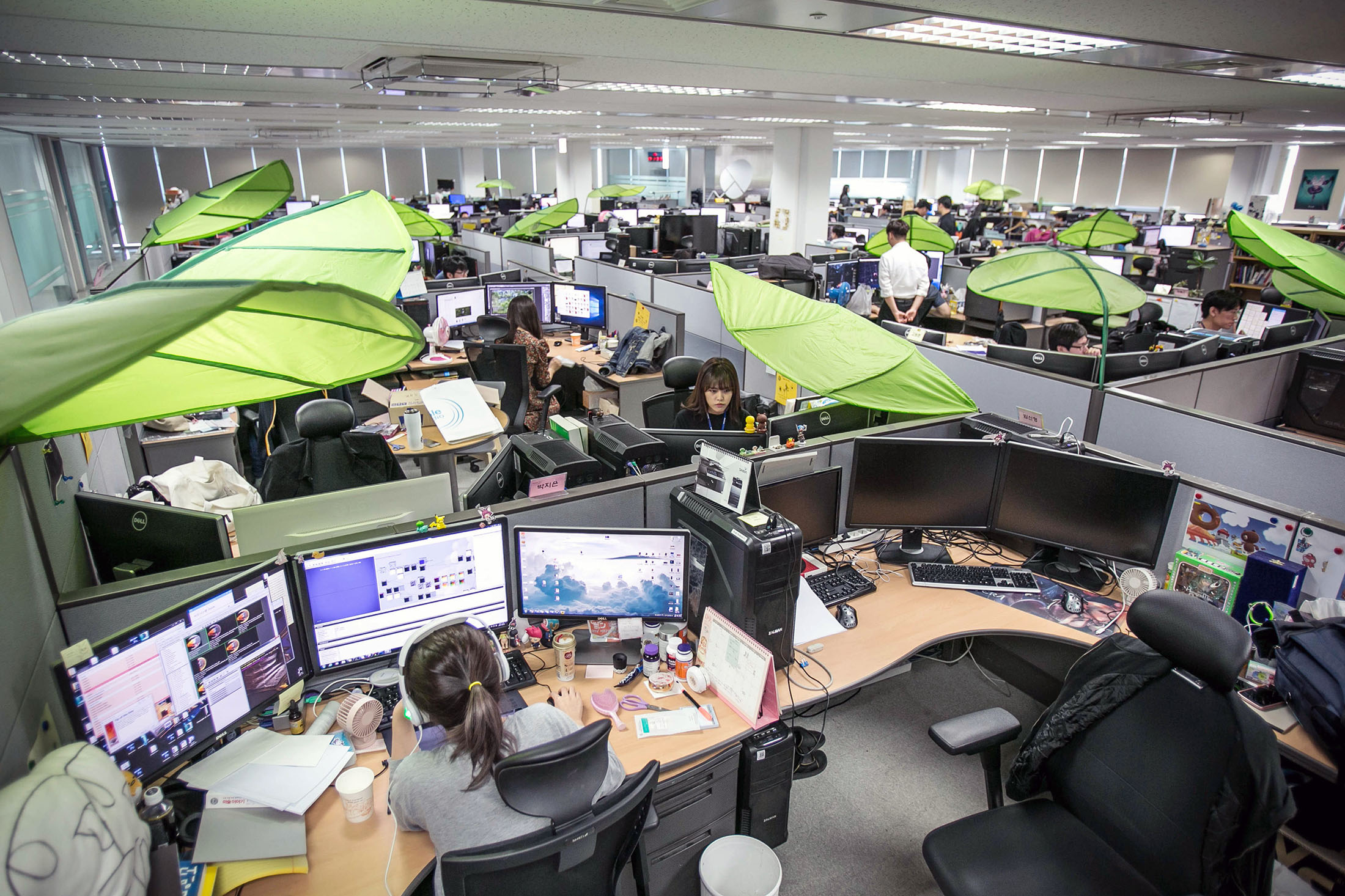The photograph depicts a vast and bustling office interior brimming with numerous gray cubicles, each densely packed with employees. Every workstation is equipped with three monitors and multiple keyboards, contributing to a scene reminiscent of an intensely busy call center. The office is illuminated by a grid of fluorescent lights on the ceiling, casting a stark and somewhat harsh brightness across the room.

Interspersed among the cubicles are large, palm leaf-shaped umbrellas suspended over certain workstations. These distinctive installations serve an unclear purpose; they might be aiming to reduce glare from the overhead lighting or ambient sunlight, dampen noise levels, or possibly signify a celebratory decor. Notably, these umbrellas aren't distributed uniformly but seem strategically placed over specific cubicles.

The scene is further characterized by its cultural homogeneity, as all visible individuals appear to be of Asian descent, diligently working amidst the sea of screens and cubicles in this enormous office environment.